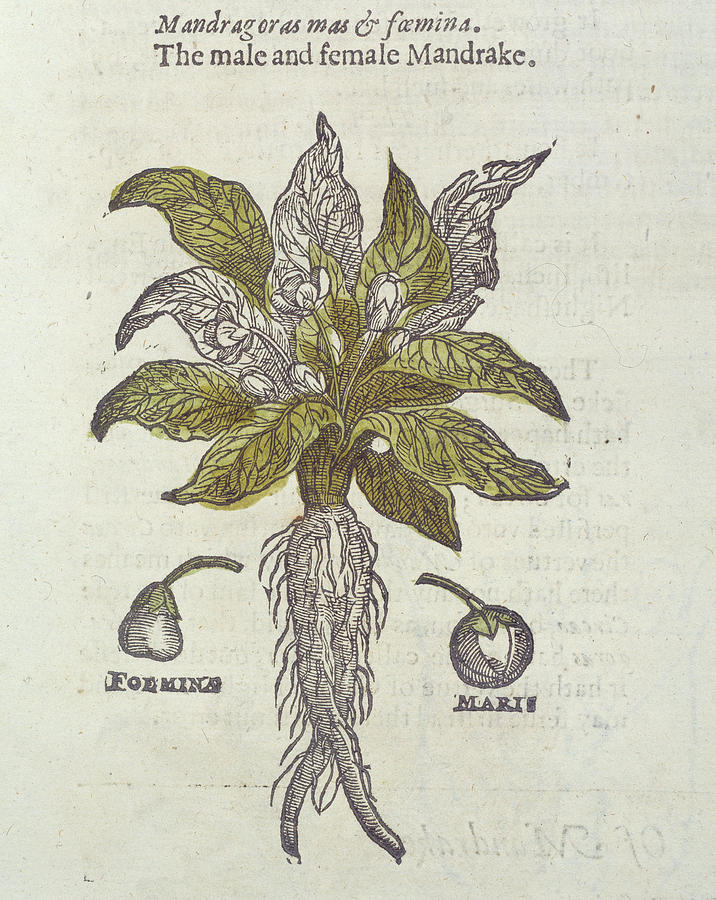This detailed drawing of a mandrake plant, appearing to be from an old botanical illustration, is set against a beige background with inscriptions in both Greek and English. Highlighting its historical essence, the top of the image features the Greek name "Mandragoras mas and femina," translating to "the male and female mandrake." Below this text, in English, it reads "the male and female mandrake." The central illustration depicts the mandrake with its prominent, large root that bifurcates almost like legs, extending upward to a thick, stocky stem.

The plant's foliage consists of green leaves, some of which are tinged with white. These leaves are detailed with a central vein and smaller veins branching out, accentuating their structure. Emerging from the center are several flower buds, some still closed while others have opened to reveal their delicate petals.

On either side of the plant, there are notable features: to the left, a small drawing resembling an acorn or pear, labeled "F-O-L-M-I-N-A," and to the right, a spherical bulb or flowering bud, labeled "M-A-R-I-S." These additional illustrations further elaborate the intricate details of the mandrake plant's anatomy.